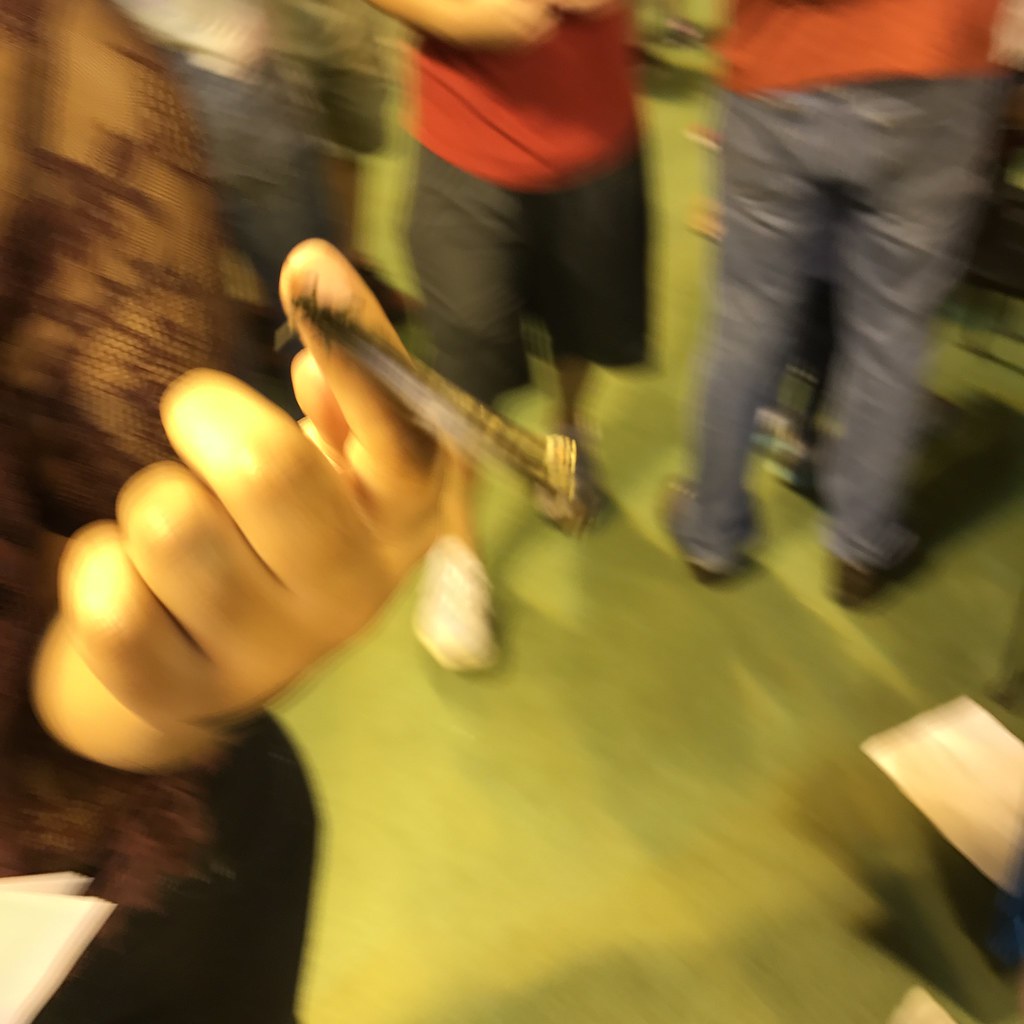A very blurry photograph captures a scene from a downward perspective, focusing on a woman's hand in the foreground. The woman, identified by her lacy top, appears to be either pointing at something or holding an object on her finger, though the motion blur makes it difficult to discern details. The ground beneath her is a greenish hue, likely due to the lighting affecting the color of the tiled surface. In the background, the lower halves of at least two other individuals are visible: one wearing black shorts with a white or red shirt, and the other dressed in jeans paired with an orange shirt.